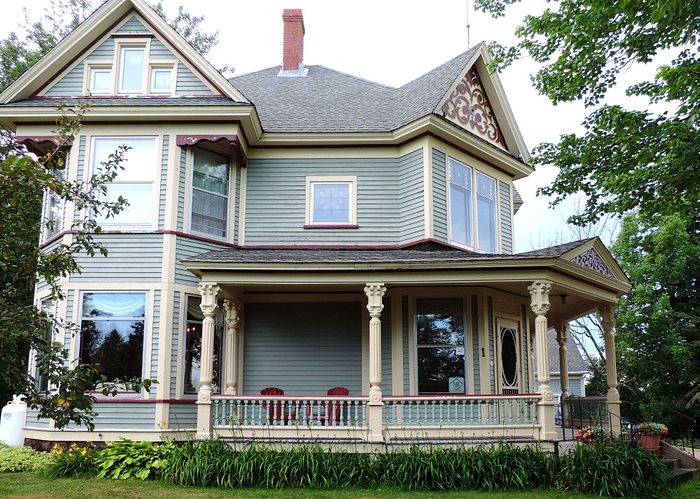The image showcases an elegant, well-maintained two-story Victorian-style home with a potential third-story walk-up attic. The house, painted in a grayish-blue hue with beige trim, features a prominent wraparound porch with intricate wood carvings on the banisters and gables. The front door, adorned with a large glass entrance, is flanked by lush landscaping which includes lilies and other blooming flowers, as well as green grasses and bushes. The porch, which extends to the right, is furnished with two red chairs and has an overhang. The roof is covered in asphalt shingles and has a red brick chimney. Windows are plentiful and detailed with shutters on some. Surrounding the house are trees on both sides, which add to the serene, picturesque setting of this thoughtfully restored home.